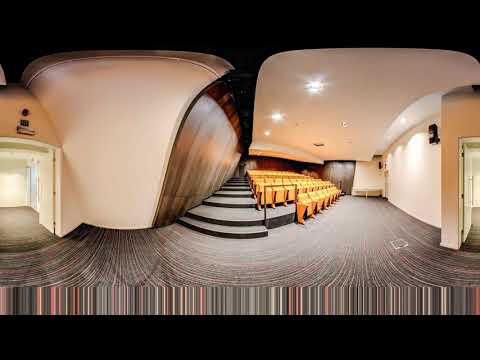This photograph captures an expansive and modernistic auditorium or theater through a fisheye panoramic view, clearly divided into two hemispheres: one on the left and one on the right. The image features black rectangular strips at the top and bottom, framing the scene. The floor of the auditorium is a gray, striped carpet with hints of red, white, and black patterns, contributing to an Art Deco aesthetic.

The walls display contrasting characteristics: the left side shows white walls curving around a wood-paneled entryway leading to a hallway, while the right side also has white walls with another entryway, suggesting multiple access points to the room. The auditorium boasts a white ceiling from which modern, white lights hang, illuminating the space with a bright, even glow.

Centrally located are rows of elevated seating, characterized by their yellowish-gold seats that are currently in their folded-up, closed positions. These seats are tiered, giving a stepped appearance, suitable for presentations or lectures. This seating arrangement hints at a lecture hall or modern presentation setup, and it's framed by a dark brown or black arch that adds to the elegant, sophisticated atmosphere of the space. No people are present, emphasizing the architectural details and layout of the auditorium.